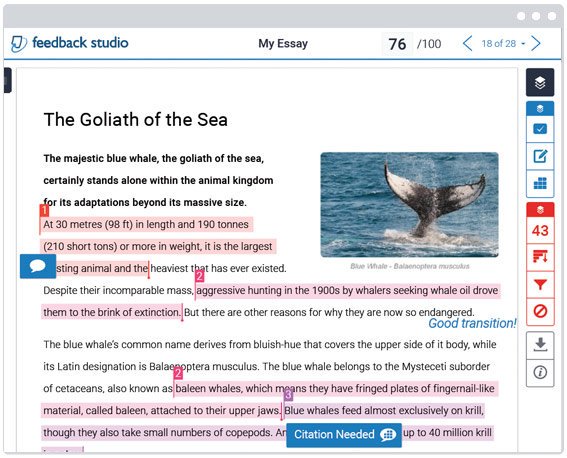The image depicts a detailed online article layout on a webpage. At the very top of the page, there is a light gray horizontal bar spanning the width of the page, occupying about one-eighth of the screen's height. Within this gray bar, three white circles are aligned in the top right corner. The rest of the webpage showcases a clean, crisp white background. 

On the left side of this header, a small blue logo is followed by the words "feedback studio" in all lowercase letters, displayed in the same blue font. Positioned centrally, the text "my essay" appears in black font. Slightly to the right of this, the text "76/100" is presented, with "76" in bold black and "100" in regular black font. Adjacent to this is a navigation element comprising a less than sign ("<"), the text "18 of 28" in blue with a pull-down menu, and a greater than sign (">").

The main section of the page begins with a bold black title, "The Goliath of the sea." Below this, in bold black font, is the opening sentence, "The majestic blue whale, the Goliath of the sea certainly stands alone within the animal kingdom for its adaptations beyond its massive size." This sentence is followed by highlighted coral-colored text detailing the whale's size: "At 30 meters (98 feet) in length and 190 tons (210 short tons) or more in weight. It is the largest..." 

A small blue rectangular overlay with a white speech bubble obscures the next word. The sentence continues, "animal and the heaviest that has ever existed." 

A white number one in a bright coral vertical rectangle precedes the highlighted section, marking the beginning of the first annotation. 

Further down, a white number two in a bright coral vertical rectangle indicates another annotation, followed by highlighted text: "Aggressive hunting in the 1990s by whalers seeking whale oil drove them to the brink of extinction." The highlighting ends here, and the text continues in regular black font: "But there are other reasons for why they are now so endangered."

Below this, in blue font, there is an encouraging comment: "good transition!"

The next paragraph begins in regular black font: "The blue whale's common name derives from the bluish hue that covers the upper side of its body while its Latin designation, musculus..." The continuation of this text is obscured by another overlay.

Another annotation marked by a white number three in a purple vertical rectangle appears along with more highlighted text: "The blue whale belongs to the mysticeti suborder of cetaceans, also known as baleen whales, which means they have fringe plates of fingernail-like material called baleen attached to the upper jaws."

Still highlighted, the text mentions, "Blue whales feed almost exclusively on krill, though they take small numbers of copepods." A horizontal blue box with white text reading "citation needed" obscures some words. The text continues with, "up to 40 million krill," but the subsequent line is cut off by the page's edge.

Adjacent to this beginning content on the left is an image displaying a horizontal view of a whale's tail emerging from the ocean. The article continues to fill the remainder of the page width, and icons are aligned vertically along the right margin.